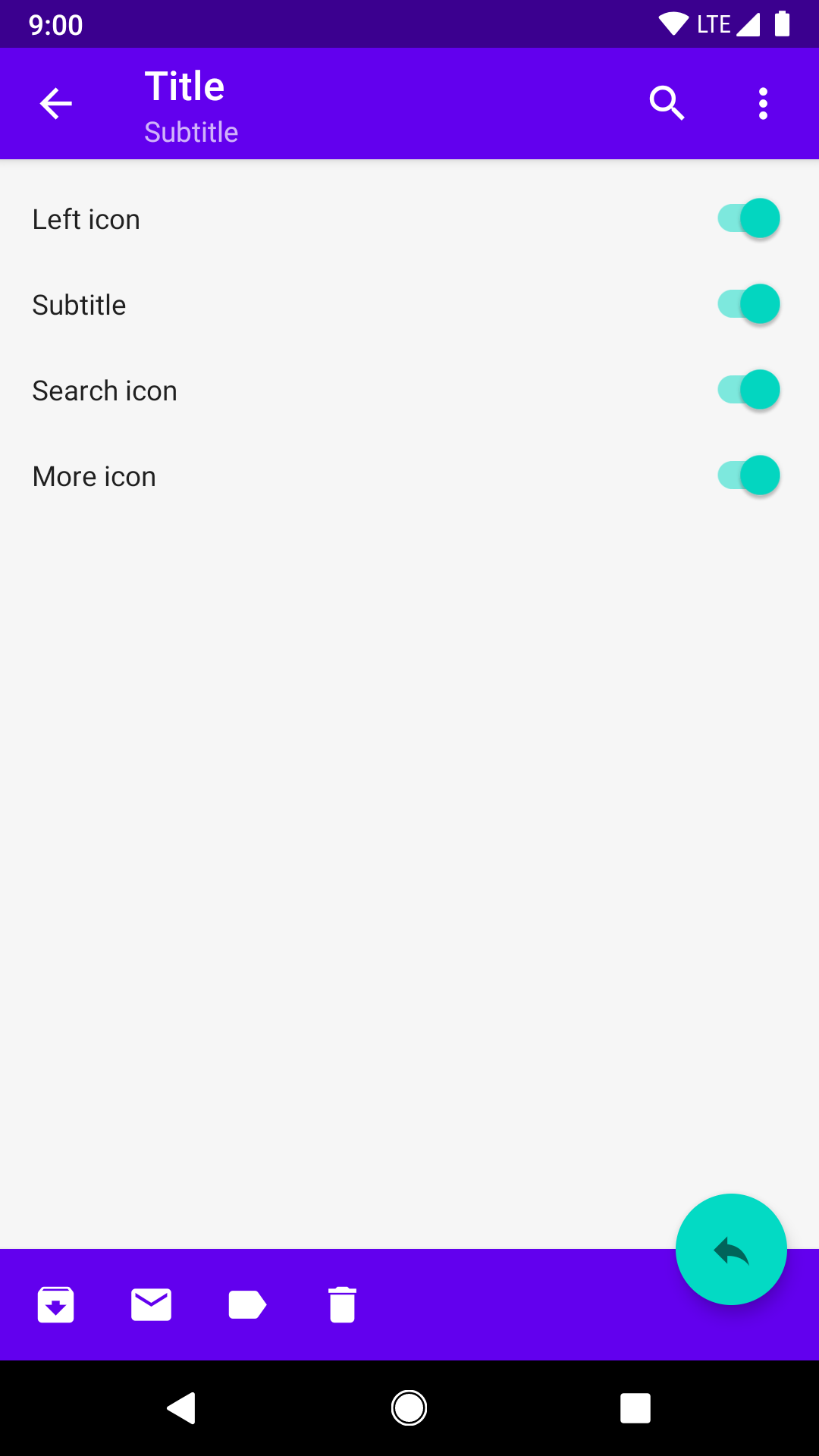The screenshot displays a settings menu with a primary background color of light gray. The accent colors used are royal blue, purple, and jade green. In the top left corner, the time is displayed in purple, reading 9 o'clock. The top right corner features a white Wi-Fi icon, followed by "LTE" in white, cellular signal bars, and a battery indicator all in white.

At the top of the screen, the header reads "Title" with "Subtitle" directly underneath it. To the right of these headings is a search icon represented by a magnifying glass. Below this header section, there are four rows of text, each accompanied by a toggle switch that is turned on, indicated by the jade color. The text for these options is in black and the options listed are "Left Icon," "Subtitle," "Search Icon," and "More Icon."

In the bottom right-hand corner of the screen, there is a jade green return icon, depicted as a left-facing arrow. Along the bottom of the screen is a blue header containing four white icons: a download icon, a message icon, a tag icon, and a trash icon.